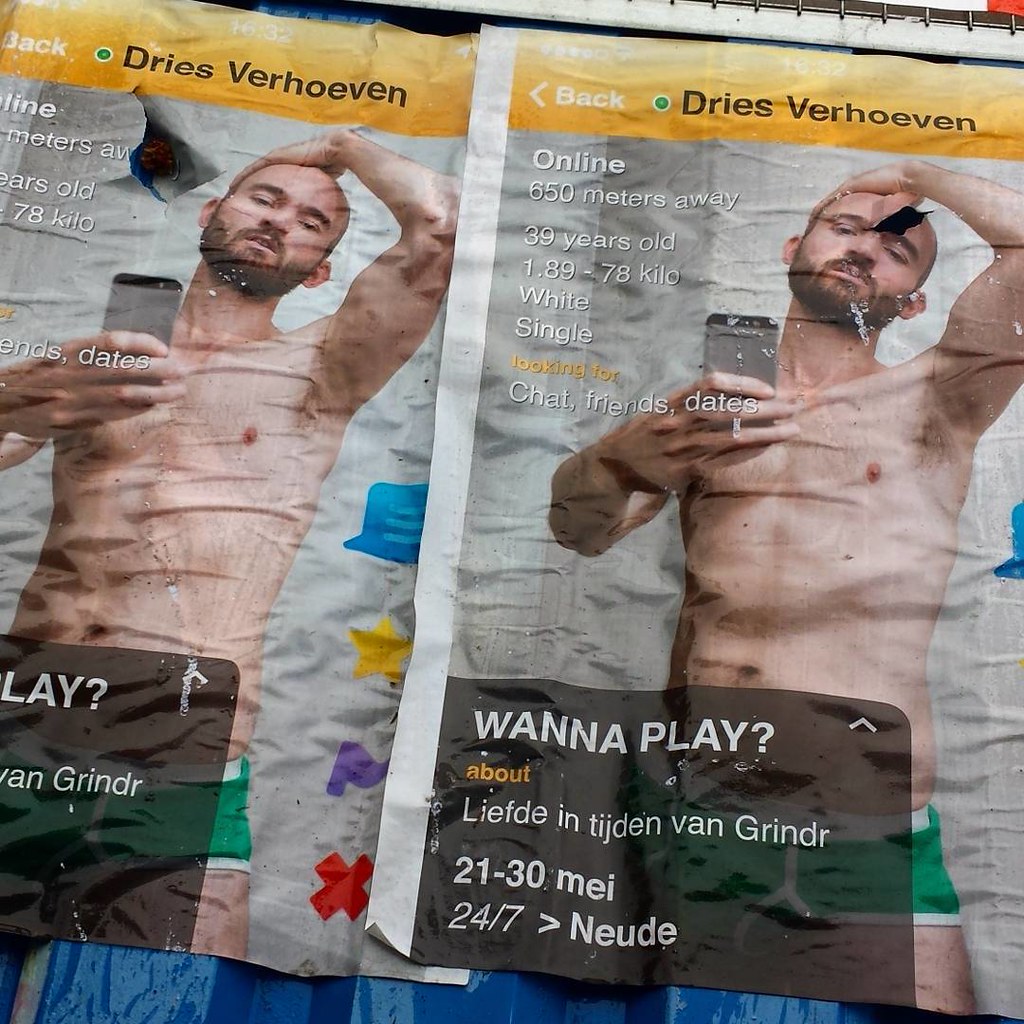The image depicts a printed screenshot from the Grindr app, capturing multiple pages of the printout. At the top, there is an orange bar with a white "back" button and the name "Gijs Verhoeven" in black font, indicating online status with a small green circle. The central figure is a middle-aged, balding man with a brown goatee, taking a selfie in the mirror while wearing only green briefs. The left-hand side of the image contains white text stating he is "online, 650 meters away, 39 years old, 1.89 meters tall, 78 kilos, white, single, and looking for chat, friends, and dates." At the bottom left, a black box reads "want to play," followed by further details including an "about" section, distance, and a note saying "24-7 nude." This descriptive profile photo appears duplicated on the right side of the printout.